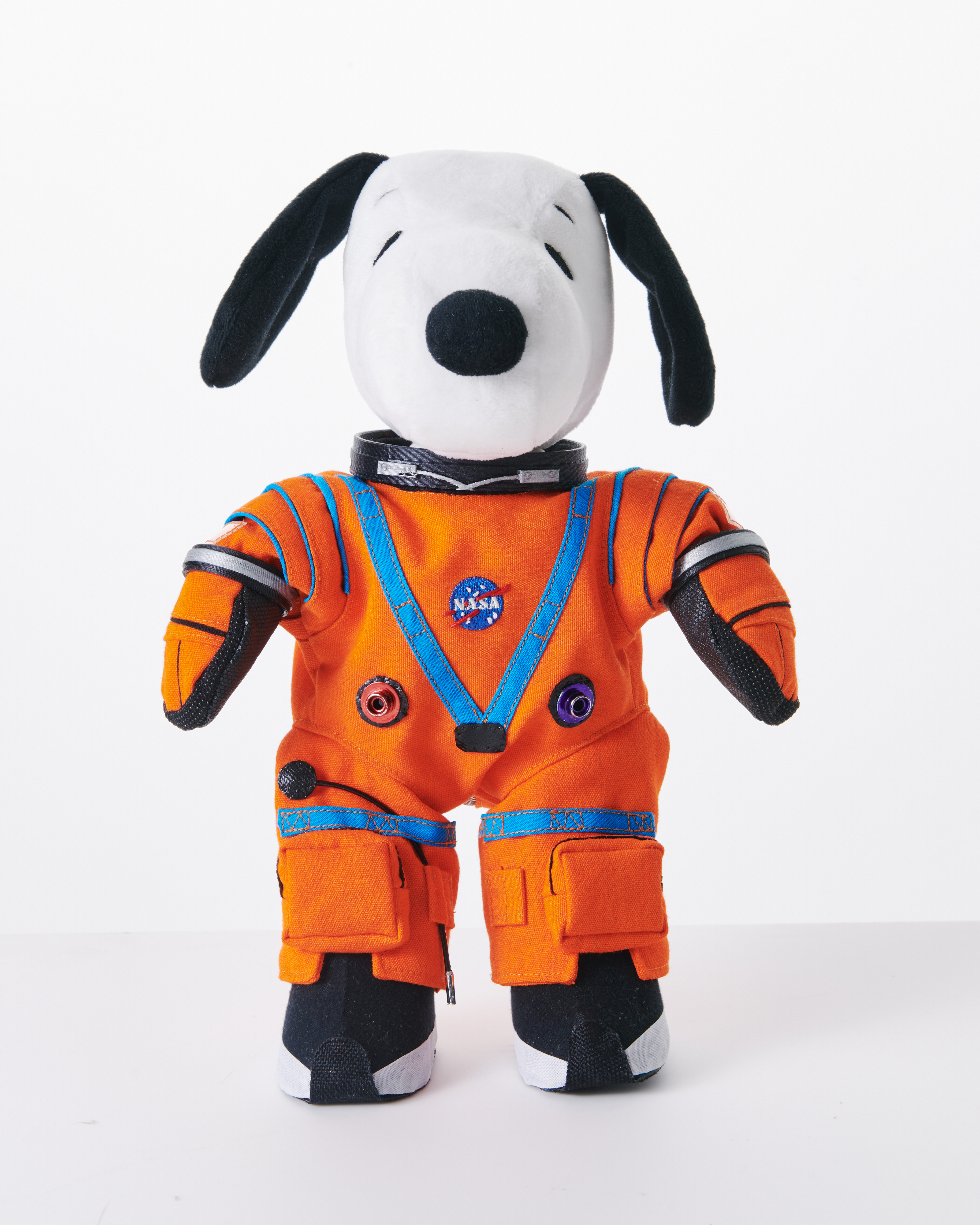The image features a Snoopy doll dressed in a bright orange astronaut suit, standing upright on a white background, likely on a white table. The Snoopy doll, which is a white dog with black ears, nose, and eyes, has its head exposed while the rest of its body is covered by the space suit. The astronaut outfit is highlighted with light blue stitching, red and blue connection ports on the chest, and a prominent NASA badge centrally located on the chest area. The suit includes orange gloves with black interiors, black and white shoes with Velcro enclosures at the ankles, and a colorful band around the neck resembling a choker, accentuating Snoopy's neck. Snoopy is standing with its arms by its sides, looking directly into the camera, adding to the overall cute and charming appearance of the photograph. Notably, the outfit does not include a helmet.